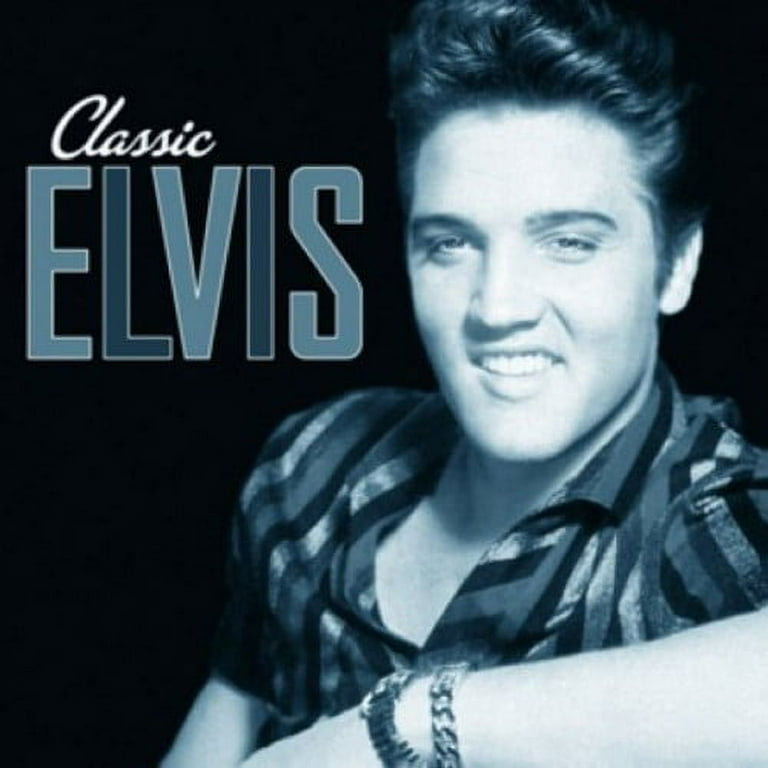The image resembles an album cover with a black background that prominently features Elvis Presley. On the left side, the words "Classic Elvis" are displayed, with "Classic" written in smaller white cursive script and "Elvis" in large, bold letters that alternate between different shades of blue and green. Taking up most of the right side of the image is a black-and-white photograph of Elvis. He is wearing a vertically striped shirt with the top button undone, revealing his throat and the upper part of his chest. Elvis is depicted from the chest up, slightly leaning on one arm, with a bracelet or watch visible around his wrist. His signature pompadour hairstyle is perfectly styled, and he gazes directly at the camera with a confident smile, exuding charisma. The detailed stripes on his shirt vary in shades of black, gray, and white, enhancing his iconic look. The image captures the essence of Elvis Presley during his prime, evoking the nostalgia of his impactful presence in music and pop culture.